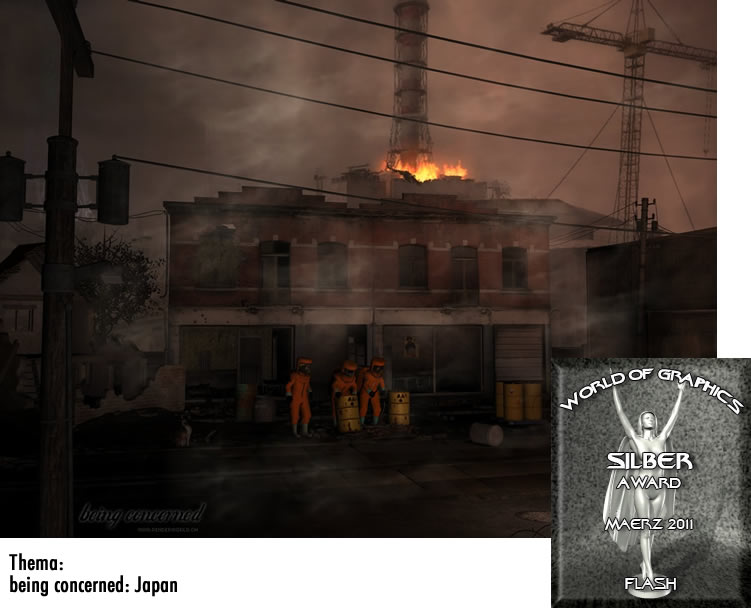The image appears to be a computer-rendered, video game-style scene with a surreal and somewhat cartoonish vibe. It features an industrial building, possibly a factory or power plant, engulfed in smoke and flames, creating an apocalyptic atmosphere. The background showcases a dark, smoky sky with visible fog and an industrial crane looming ominously. In the foreground, three individuals in orange hazmat suits are handling yellow barrels marked with hazard symbols, likely indicating toxic or radioactive materials. Scattered around are more hazardous barrels, intensifying the scene's hazardous environment. An adjacent award plaque, placed in the bottom right corner, displays "World of Graphics, Silver Award, Mayer's 2011" with an image of a silver woman raising her arms and wearing a flowing silver cape, symbolizing a trophy. On the bottom left, black text reads "FEMA being concerned, Japan," adding a layer of context to the disaster depicted. The overall composition suggests a catastrophic event with emergency personnel attempting to manage the crisis.